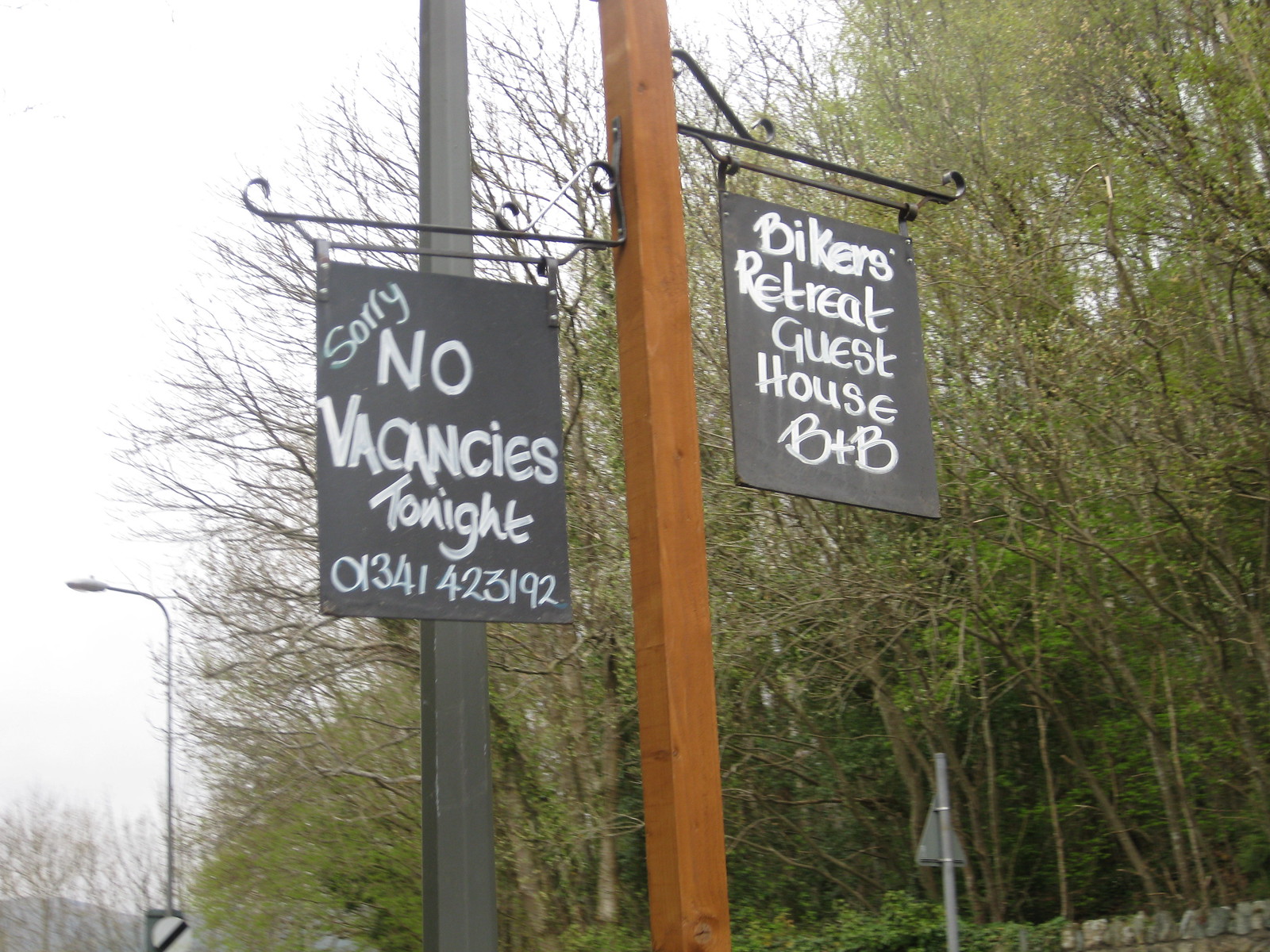This outdoor photograph features a detailed scene centered around a wooden signpost with black metal rods mounted horizontally from it, holding two prominent chalkboard-style signs. The left sign reads, "Sorry, no vacancies tonight," followed by a phone number "01341 423192." The right sign advertises, "Bikers Retreat Guesthouse B&B." This signpost, stained dark brown, stands next to a gray streetlight post. The backdrop showcases a gray, overcast sky and a stone wall on the bottom right, beyond which tall, green trees line a pathway or road. The overall ambience is quite drab, with muted tones of gray and brown, except for the vibrant black and white signage that stands out in the foreground. There are additional lamp posts and scattered signage contributing to the scene.